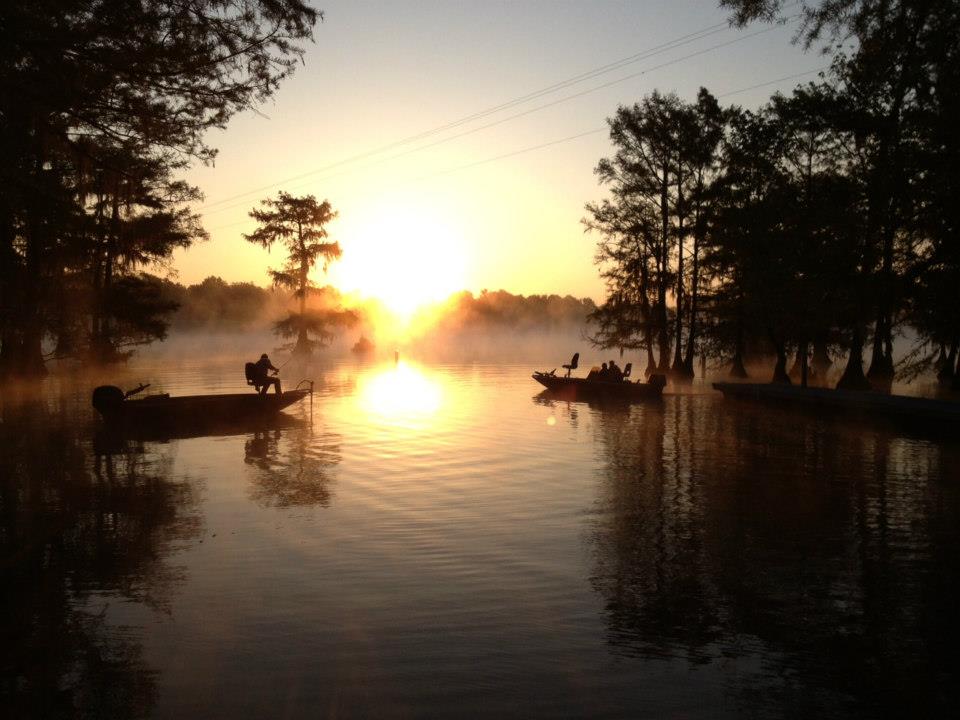A serene real-life photograph captures the Sun setting over a picturesque lake. The lake dominates the foreground, occupying the lower half of the image, and as it stretches into the distance, it meets a landscape that could be hills or clusters of trees. A soft fog veils the lake's surface in front of this natural backdrop, adding an ethereal quality to the scene. The setting Sun, a bright yellow circle, descends behind the central cluster of trees, casting radiant beams that reflect vividly on the tranquil waters below.

At the center of the image, a silhouette of a person can be seen seated in a small motorboat, designed to accommodate no more than two or three people. The Sun's powerful glow creates stark silhouettes of objects and people in the water, rendering elements into dark shapes. To the right, another silhouette appears, which could be another boat or perhaps objects closer to the tree-lined shore. This area also features visible chairs, their exact positioning ambiguous due to the interplay of light and shadow.

The lake mirrors the silhouetted trees on both sides, which frame the scene with their dark outlines. Adding a subtle detail, thin electrical wires stretch across the image from the upper left to the top right, cutting across the tops of the trees at a diagonal. Despite their delicate appearance, these wires contribute to the overall composition of this tranquil sunset moment.